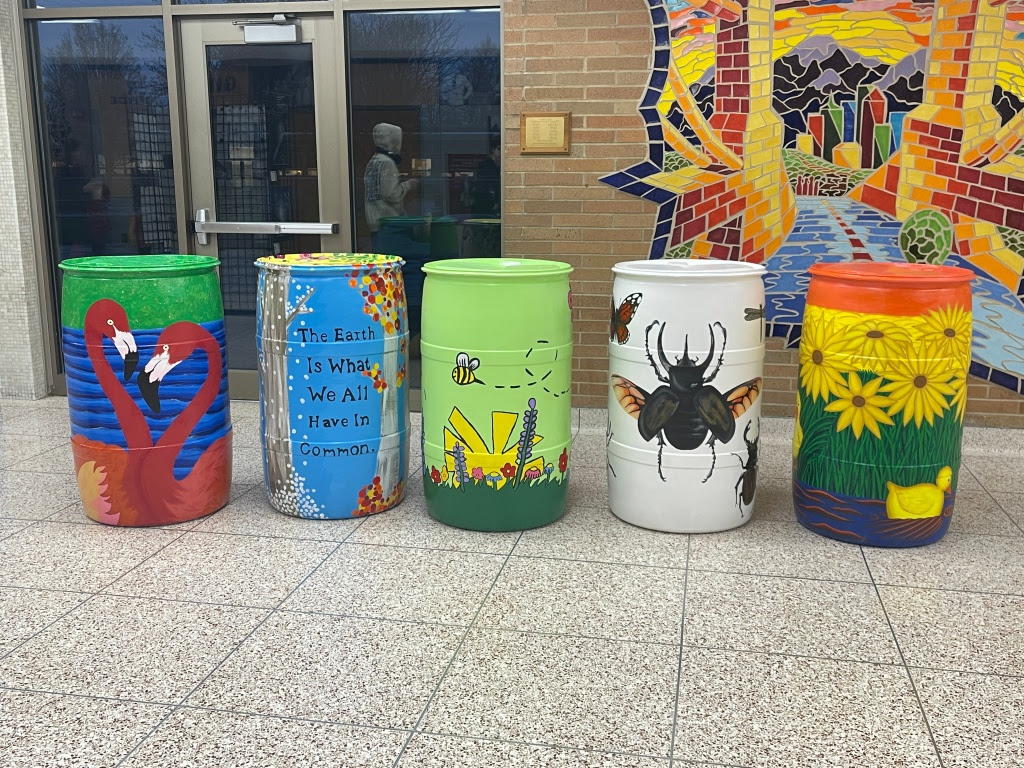The image depicts the front exterior of a brick building featuring a push-open door flanked by two large glass windows. Visible through the glass door is a woman standing near a counter, presumably a reception desk. The building's brick wall is adorned with a colorful mural that depicts a pathway leading to a cityscape with varying colors, black mountains, and a sunset.

In front of the building, the tiled sidewalk, made up of white square tiles with brown polka dots, showcases five prominently painted barrels, each approximately 55 gallons in size. Starting from the left, the first barrel is adorned with vibrant pinkish-red flamingos against a blue middle section and a green top. The second barrel hosts the phrase "the earth is what we all have in common" set against a background that includes a sky and trees. The third barrel is lime-green, featuring a flying bee on a sunny green field. The fourth barrel, white, is decorated with various insects, including butterflies and moths. The final barrel, with an orange top and blue bottom, depicts a scene of sunflowers and includes a small duck floating on a lake.